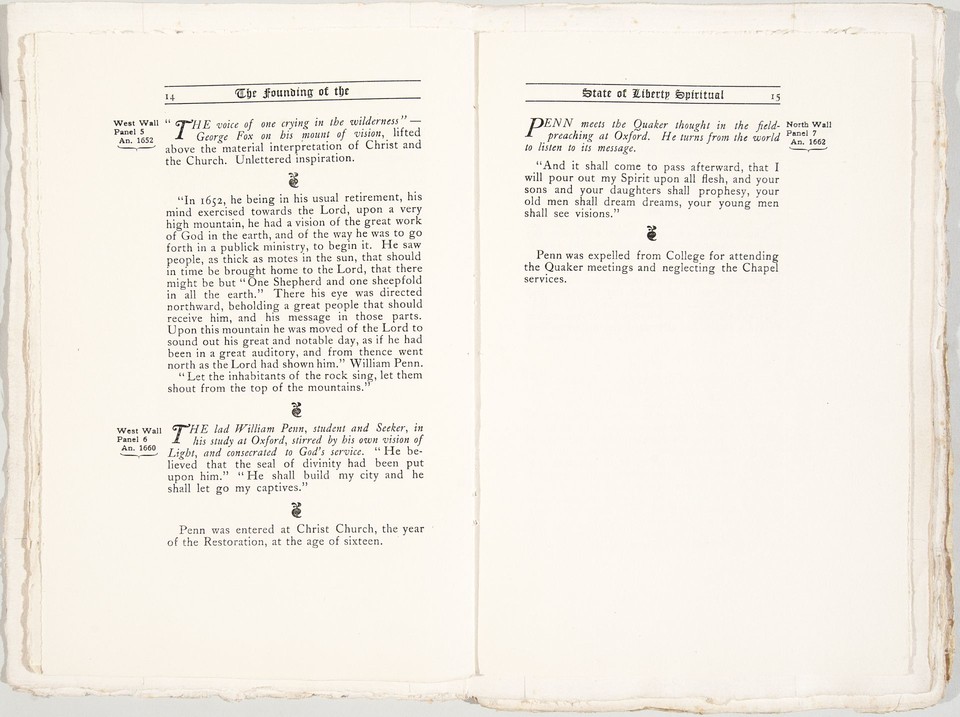The image depicts a clear and bright photograph of an open book turned to pages 14 and 15, illuminated by ample natural lighting. The book appears to be an old manuscript, featuring off-white, slightly worn pages with black text. The left page, numbered 14, prominently displays the heading "The Founding of the" and includes multiple paragraphs of text, interspersed with small black symbols resembling turnips. At the bottom of this page, it mentions "West Wall, Panel 5, AN 1652" and "West Wall, Panel 6, AN 1660." The right page, numbered 15, is titled "State of Liberty, Spiritual" and contains three paragraphs of text, similarly separated by the turnip-like symbols. This page also references "North Wall, Panel 7, AN 1662." The text on page 15 begins with "The Voice of One Crying in the Wilderness," and discusses George Fox and his spiritual insights. Overall, the manuscript's content delves into historical and spiritual themes, possibly related to the founding principles of liberty and spirituality.